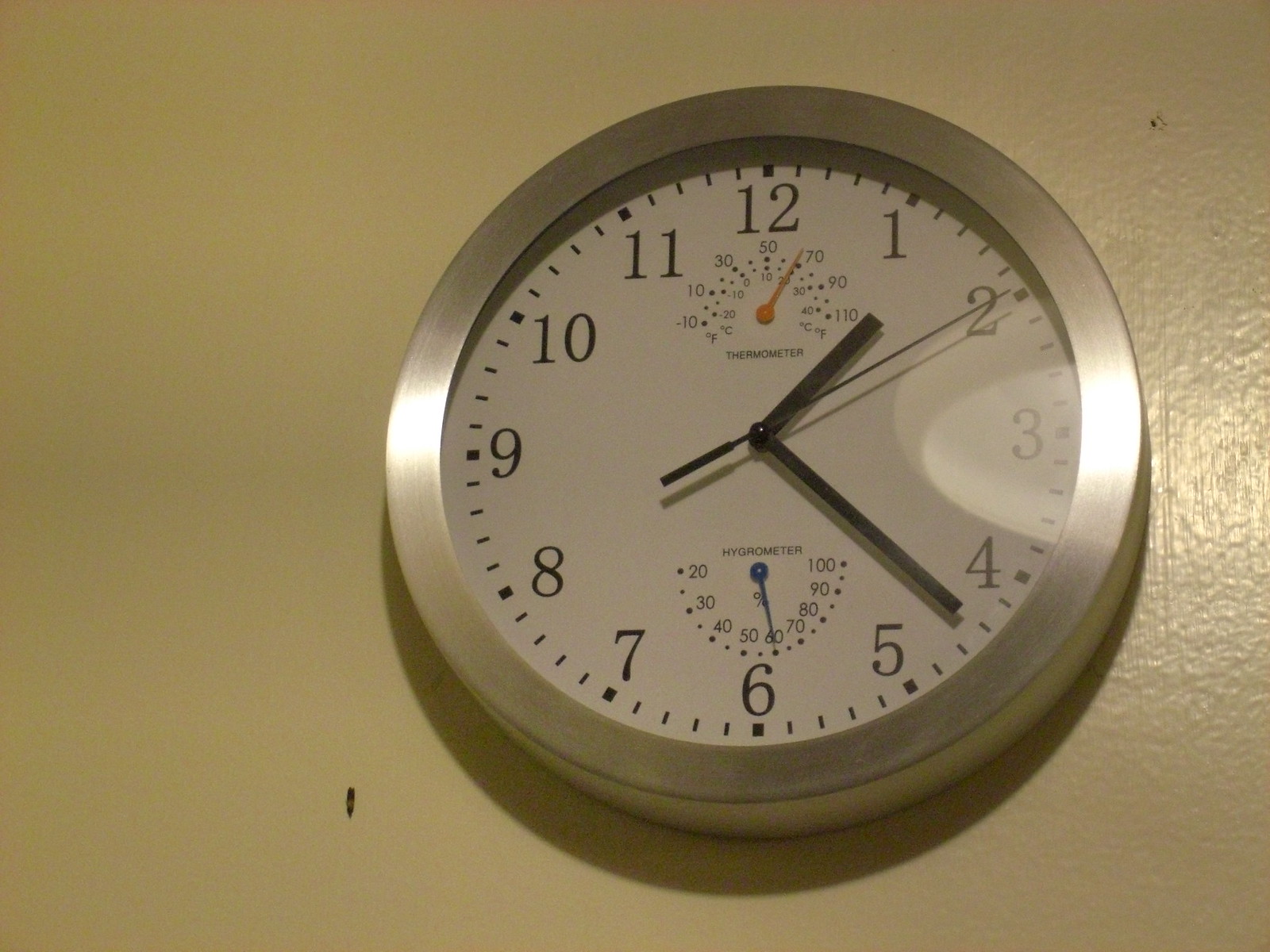A detailed photograph showcases an analog clock mounted on a cream-colored wall. This standard timepiece features a white face adorned with the numbers 1 through 12, encircled by a sleek silver border. The black hands of the clock indicate the current time as 1:22:10. This multi-functional clock also includes a hygrometer and a thermometer. The hygrometer, distinguished by a percentage symbol, registers the humidity at approximately 61%. Meanwhile, the thermometer measures the temperature at about 20 degrees Celsius, equivalent to around 68 degrees Fahrenheit. This comprehensive depiction provides a clear and informative view of the clock's features and its surrounding environment.